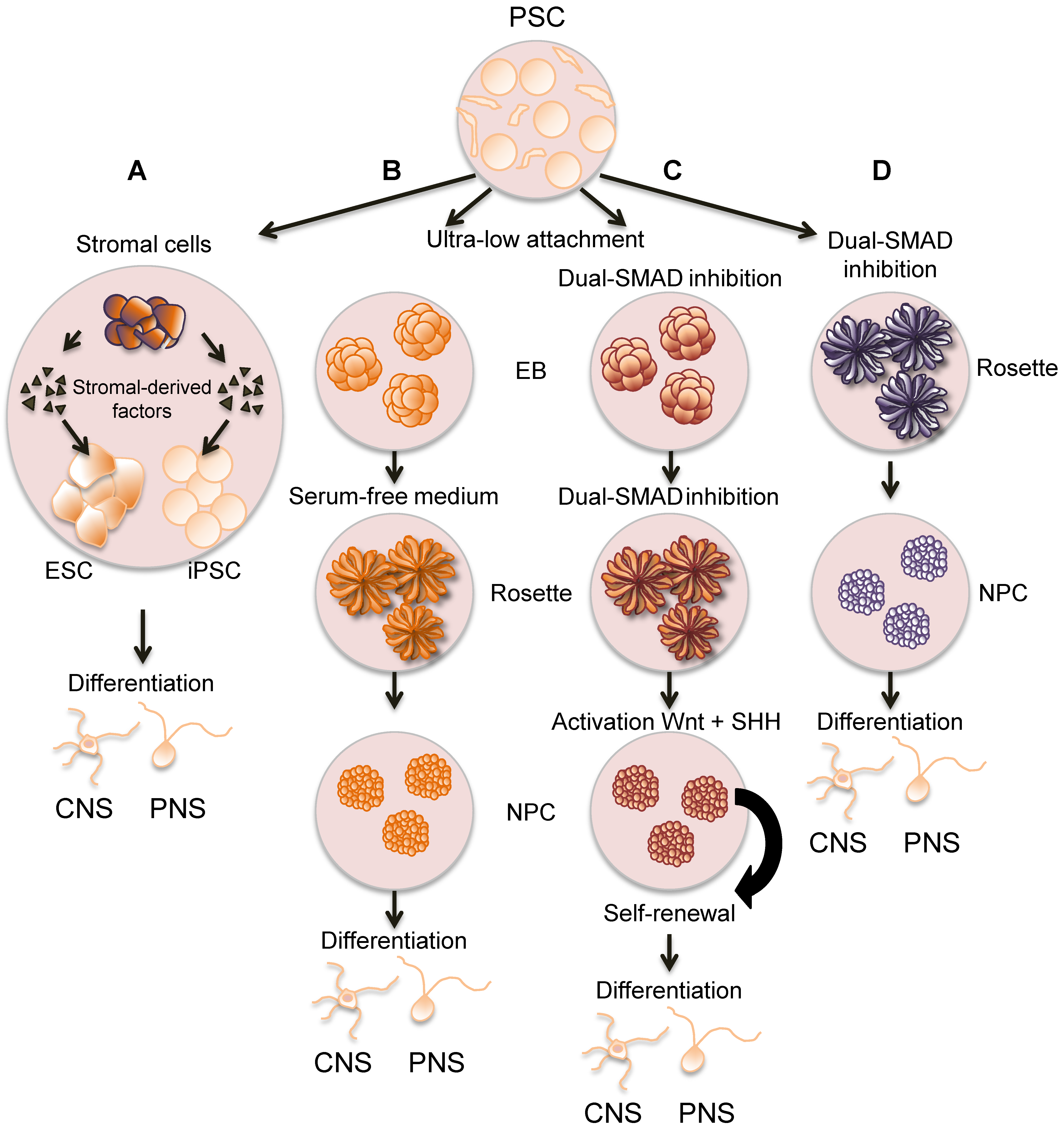The image is a detailed diagram set against a white background, featuring a central peach-colored circle at the top labeled "PSC" which stands for pluripotent stem cells. This circle contains several light pink dots and is connected by arrows to four vertical columns, each signifying a different method or pathway for cell differentiation. The arrows in these pathways are labeled A, B, C, and D.

Column A highlights "stromal cells" and "stromal-derived factors," leading to "ESC, IPSC," and includes stages of "differentiation" towards "CNS" and "PNS." Column B describes the pathway involving "serum-free medium," also ending in "differentiation" towards "CNS" and "PNS." Between columns B and C, there are labels for "EB," "Rosetta," and "NPC."

Column C emphasizes the technique "dual-SMAD inhibition," mentioning both "activation" and pathways involving "WNT" and "SHH" that lead to "self-renewal" and subsequent "differentiation" to "CNS" and "PNS." Similarly, column D repeats "dual-SMAD inhibition" and details stages involving "Rosetta," "NPC," and "differentiation," culminating in "CNS" and "PNS."

Each column is decorated with illustrative circles indicating various stages or factors in different shades of light pink, orange, brown, and blue, providing a comprehensive visual representation of the processes guiding stem cell differentiation.